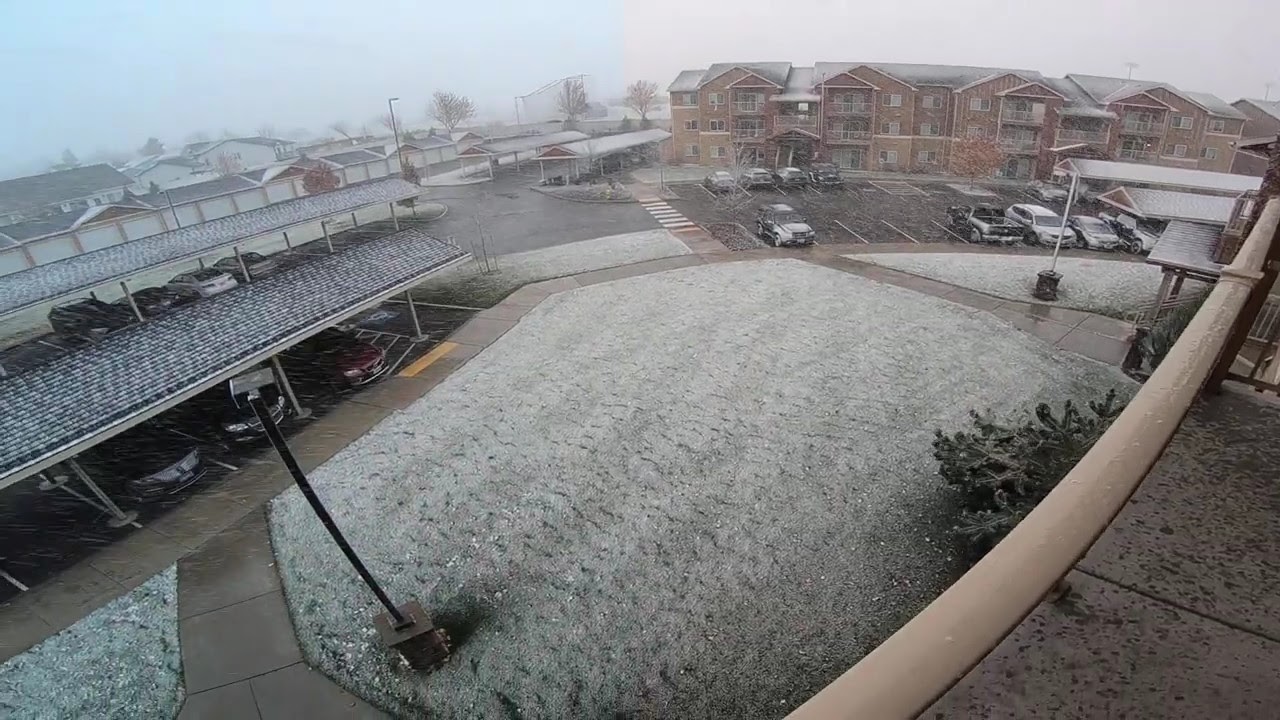The image depicts an urban parking lot on a snowy day, taken from an elevated vantage point. The parking lot, which appears to be associated with nearby buildings, is about half full, mainly with black and white cars. To the left, there is covered parking with roofs housing additional black cars. In the background, there are brown brick buildings, likely apartments or hotels, standing around three stories tall. On the far left, white houses with gray roofs are visible in the distance. Snow is lightly coating the ground, bushes, and some parked cars, indicating it has recently begun snowing. This snowfall has turned the sky a whitish-gray hue. A beige ledge and stone patio can be seen in the foreground where the photographer captured this scene. Additionally, a carport, accommodating around half a dozen cars across two levels, is situated on the left. To the right of the parking lot, a series of townhomes with balconies and white garages are aligned. In the middle of the snowy area, a light pole stands amidst scattered snow and bushes, further adding to the detailed urban winter landscape.